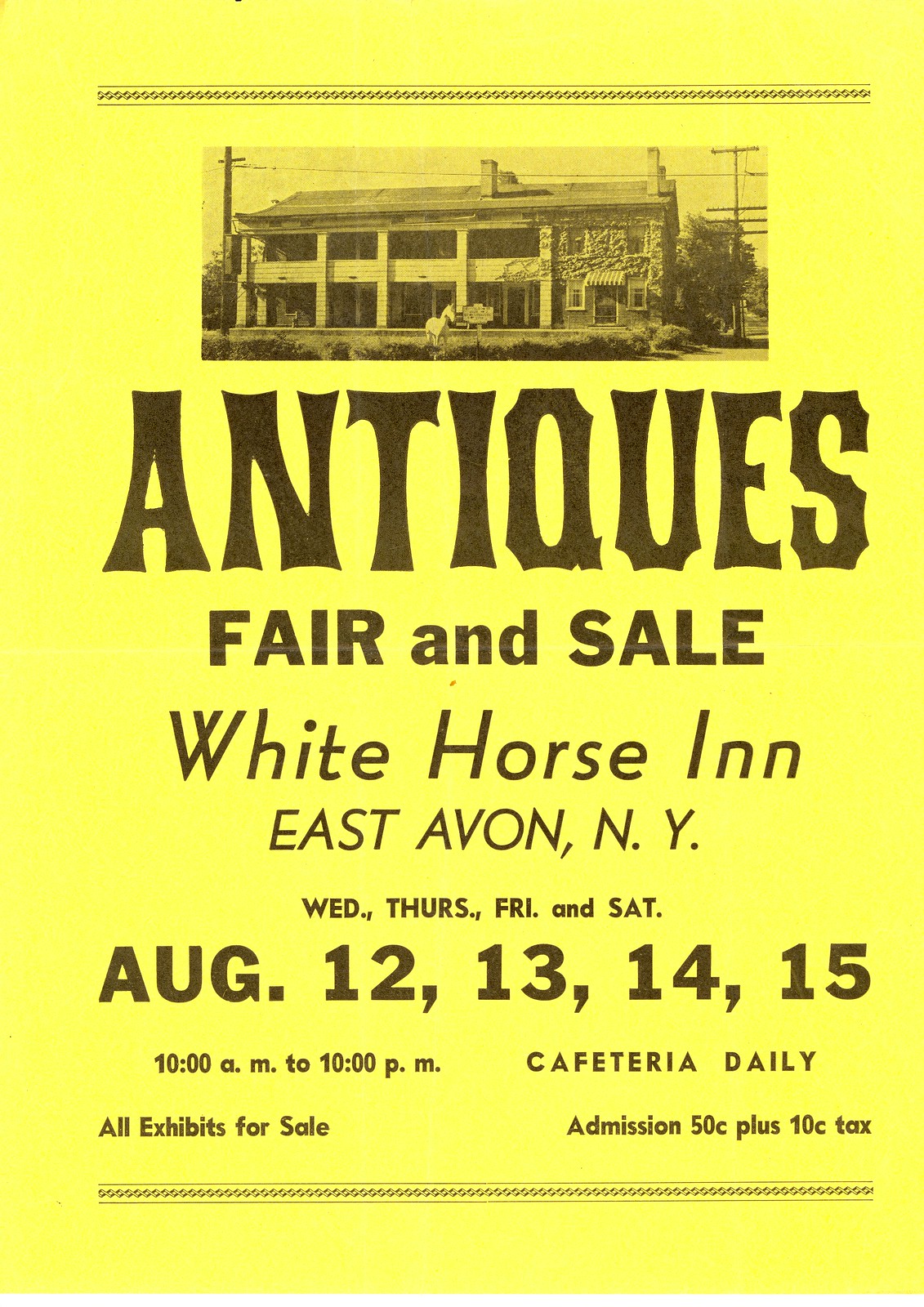This is a flyer for an antiques fair and sale, featuring a bright yellow background with dark gray text and images. At the top and bottom of the flyer are decorative brownish bars. Below the top bar is a sepia-toned photograph of the White Horse Inn, a historic two to three-story building with a horse in the front, a historical plaque, power lines, and trees. Beneath the photograph, in large black lettering, it reads "Antiques Fair and Sale," followed by smaller text indicating the location: White Horse Inn, East Avon, New York. The event is scheduled for Wednesday, Thursday, Friday, and Saturday, August 12th, 13th, 14th, and 15th, from 10 a.m. to 10 p.m. daily. A cafeteria will be open each day, and all exhibits are available for purchase. Admission is priced at $0.50 with an additional $0.10 for tax.